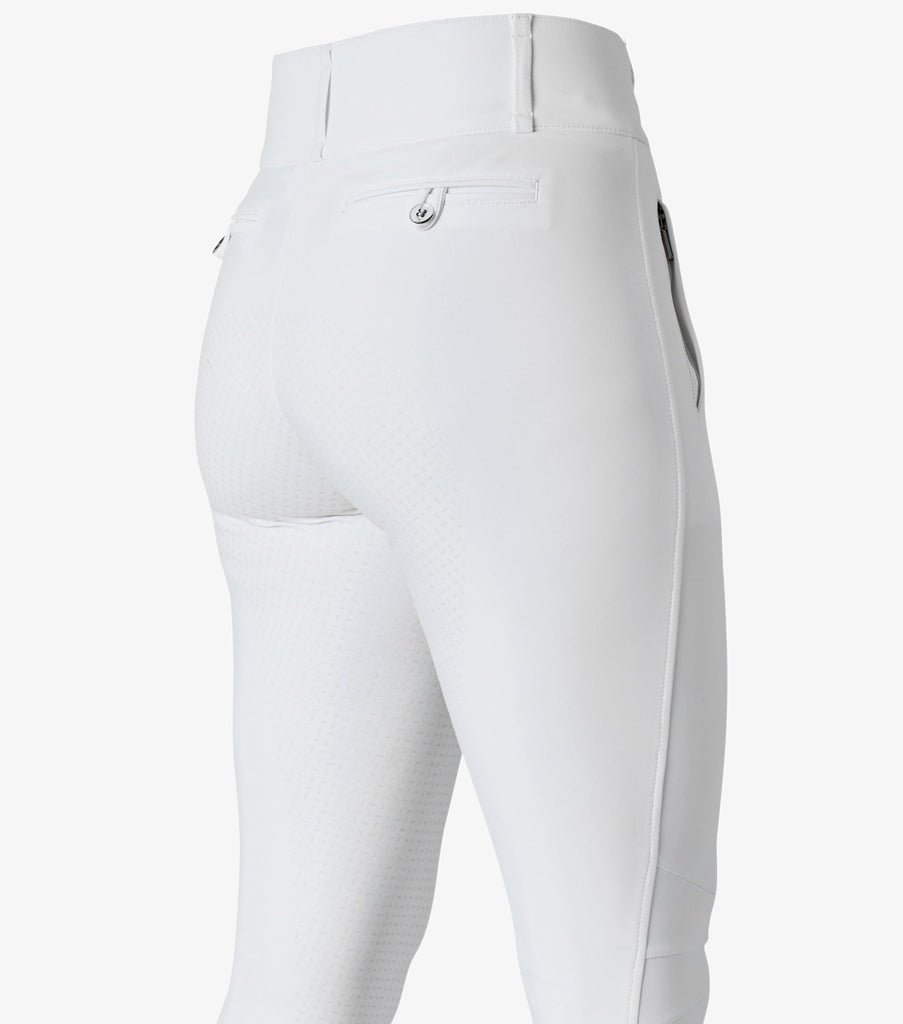This image showcases a detailed close-up side and back view of a pair of white pants that appear to be made from a specialized textured fabric, potentially a blend of cotton and rayon for a slight stretch and snug fit. The pants feature well-defined contouring around the hips and thighs, suggesting they are tailored for both aesthetic appeal and functionality, possibly intended for sports or active wear. A silver metallic button secures the waistband, which includes a visible band or belt loop. There's a small pocket with a metallic zipper closure on the right-hand side, matching the button. The design also includes wide belt loops and back pockets. Particularly notable are the light gray shadows cast across the white fabric, giving a subtle multi-tonal effect. The stitching is straight, although the seam shows some twisting and straightening. The background of the image is light gray, emphasizing the pants' detailing. The overall presentation highlights both the craftsmanship and practical features of the garment.